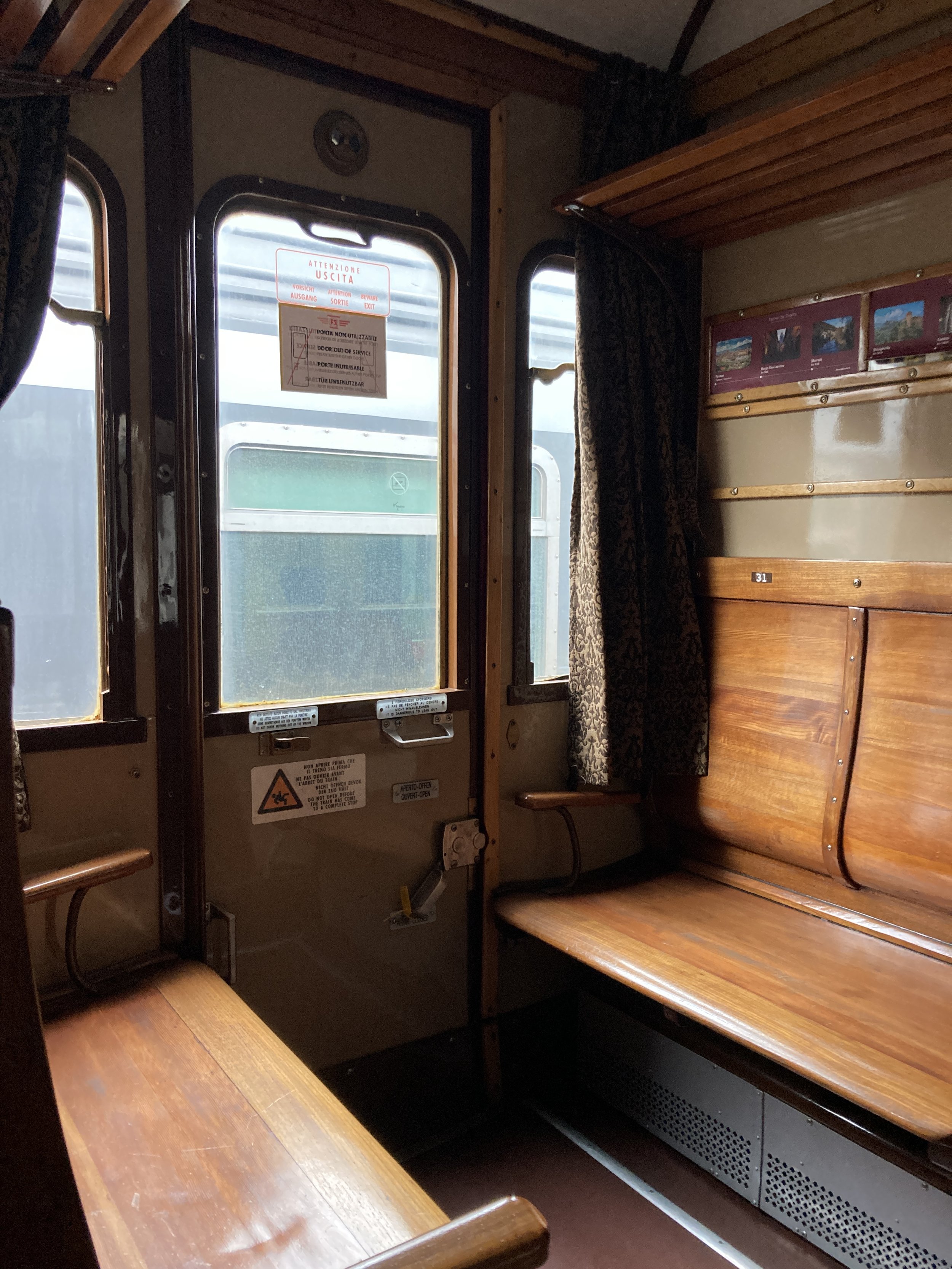The image is a detailed photograph captured inside a stationary passenger train cabin, likely an Italian model. The cabin features two wooden bench seats facing each other, designed with brown wood frames and armrests at the far ends. Bright daylight streams through the cabin's windows, illuminating the beige-colored wall behind one of the benches, which also has a wood shelf above it. The focal point of the image is a metal door at the far end of the cabin, potentially an emergency exit, featuring a large window with side windows partially covered by small curtains. The door bears Italian writing on the label and a caution regarding slipping and falling. The overall ambiance of the cabin is old-fashioned, cozy, and distinctly illuminated by natural light, making it a unique and evocative space within the train.